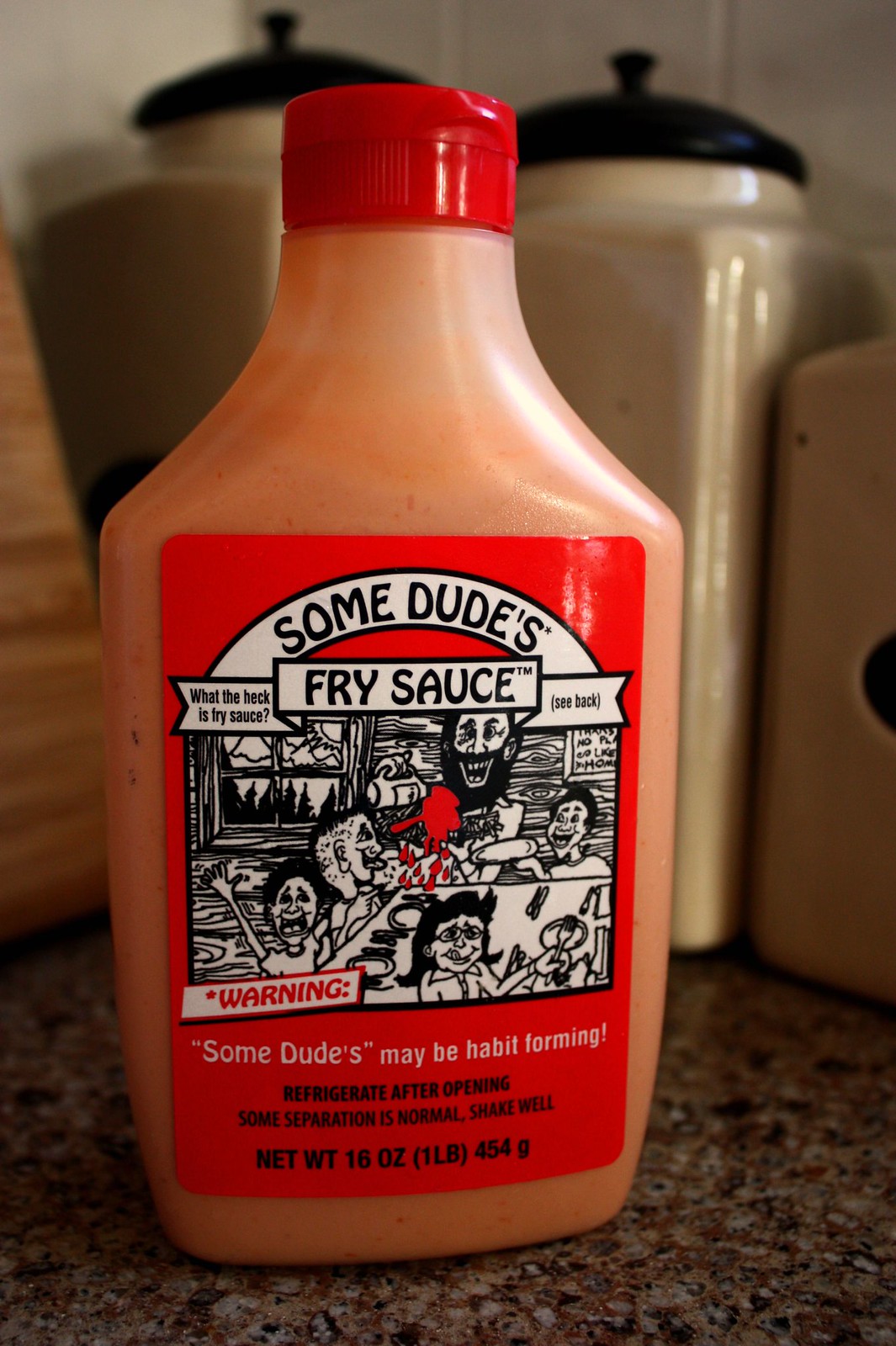This image depicts a bottle of "Some Dude's Fry Sauce" prominently placed on a kitchen counter. The bottle, which is made of semi-translucent milky plastic, reveals an orange-red liquid inside. It has a red cap and features a striking red label. The label is decorated in black, white, and red colors and shows several individuals with exaggerated expressions, suggesting excitement and enjoyment. A woman holding a spatula is among them. The label includes multiple inscriptions: "Some Dude's Fry Sauce," a playful warning that "Some dudes may be habit-forming," instructions to "Shake well" and "Refrigerate after opening," and notes that some separation is normal. The bottle's weight is listed as 16 ounces. In the background, there are three beige canisters with black lids, likely for storing kitchen staples like flour and sugar, further suggesting that the scene is set in a typical home kitchen.